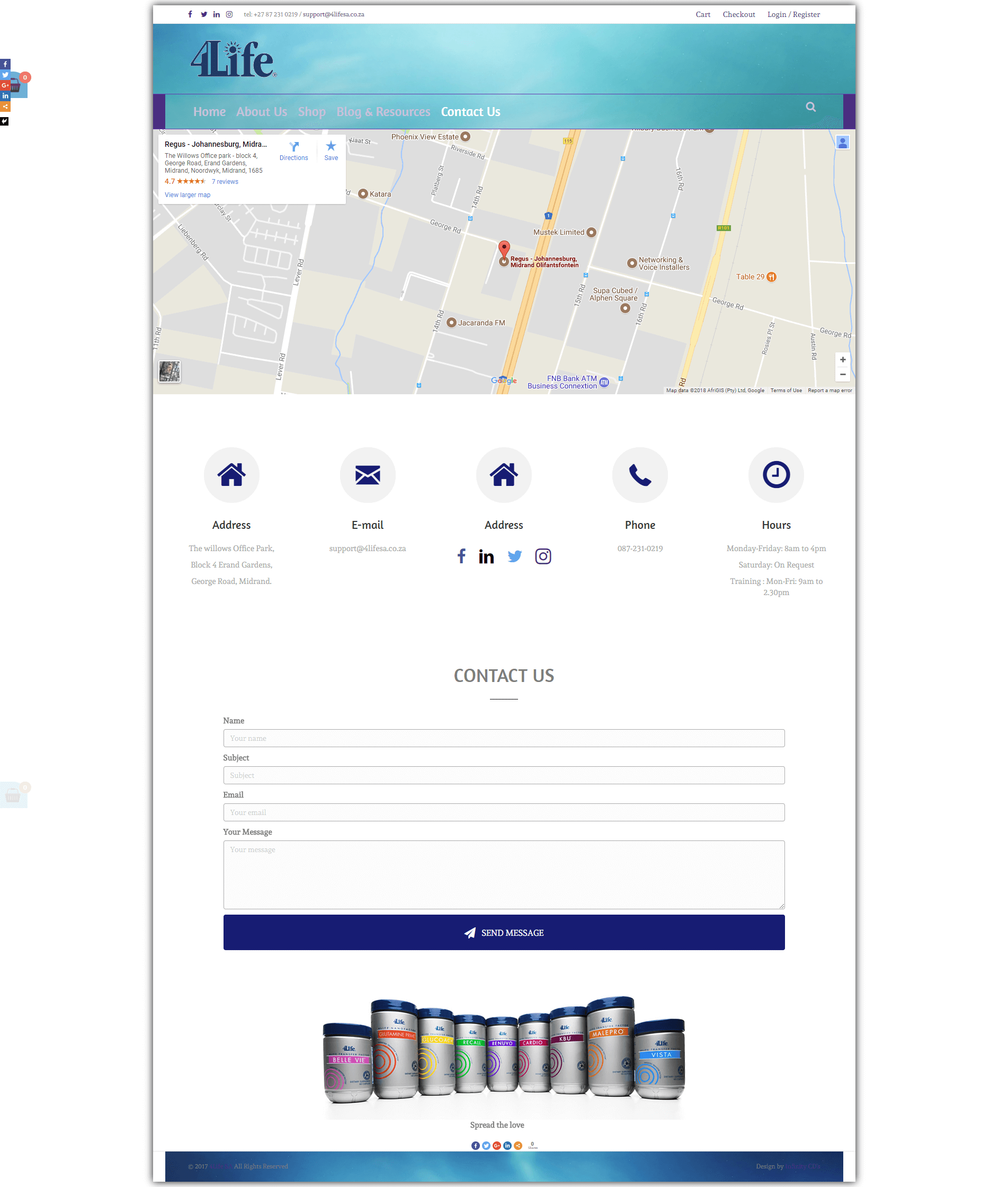This image is a screenshot of the Contact Us page from the health website titled "For Life." The navigation menu at the top indicates that the Contact Us section is highlighted in white, confirming the page's purpose. At the top of the page, there is a detailed map showcasing the company's location, alongside the listed address. Below the map, there are various icons representing the company's contact details: a location pin for the address, an envelope for email, a phone icon for contact number, and a clock to show business hours. 

Adjacent to these details are social media icons for LinkedIn, Facebook, Instagram, and Twitter, offering different ways for users to connect with the company. The page also features a Contact Us form, which includes fields for the user to input their name, subject, email, and message, complemented by a Send Message button for submissions.

At the bottom of the page, there is an image displaying several "For Life" products arranged in silver, round containers with colorful labels. These labels are red, yellow, and green, suggesting a line of health-related products, which appear to include protein powders and supplements. This comprehensive page helps users connect with the company, access social media channels, and gain insight into the product offerings.